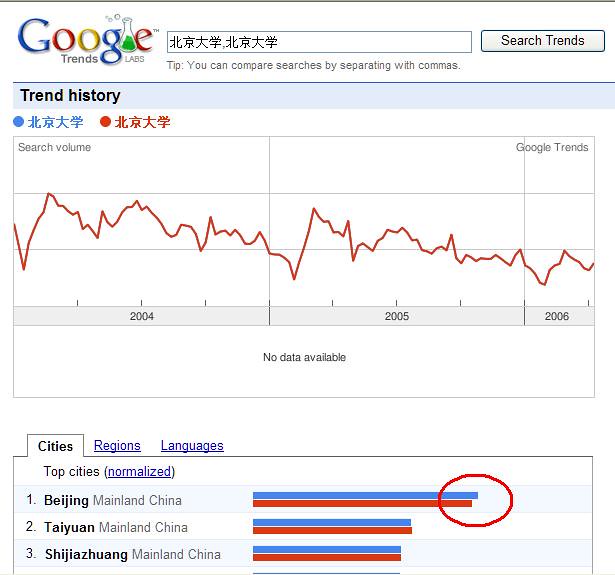The image is a detailed screenshot of a Google Trends Labs page. In the top left corner, the Google logo features stylized letters with the standard 'G' and 'G' in blue, the first 'O' in red, the second 'O' in yellow, and the 'E' in red, with the 'L' replaced by a green-filled beaker. Below the logo, it reads "Trends Labs." To the right is a search bar containing Chinese characters. Beneath this bar is a title in black font reading "Trend History" set against a light blue background.

The central part of the image displays a line chart titled "Trend History," marked with the years 2004, 2005, and 2006. The red line graph fluctuates up and down in a zigzag pattern, showing a general trend towards the right. Below the chart, in light gray lettering, it reads "Search volume," and underneath, there is a notice, "No data available."

At the bottom, a section is labeled "Top cities, normalized," displaying a list of cities including Beijing, Taiwan (actually Taiyuan), and Shijiazhuang, all identified as part of mainland China. Accompanying the city names are bar charts featuring red and blue bars, with blue on top. Beijing has the longest bars, and there is a red circle at the end of its bar graph.